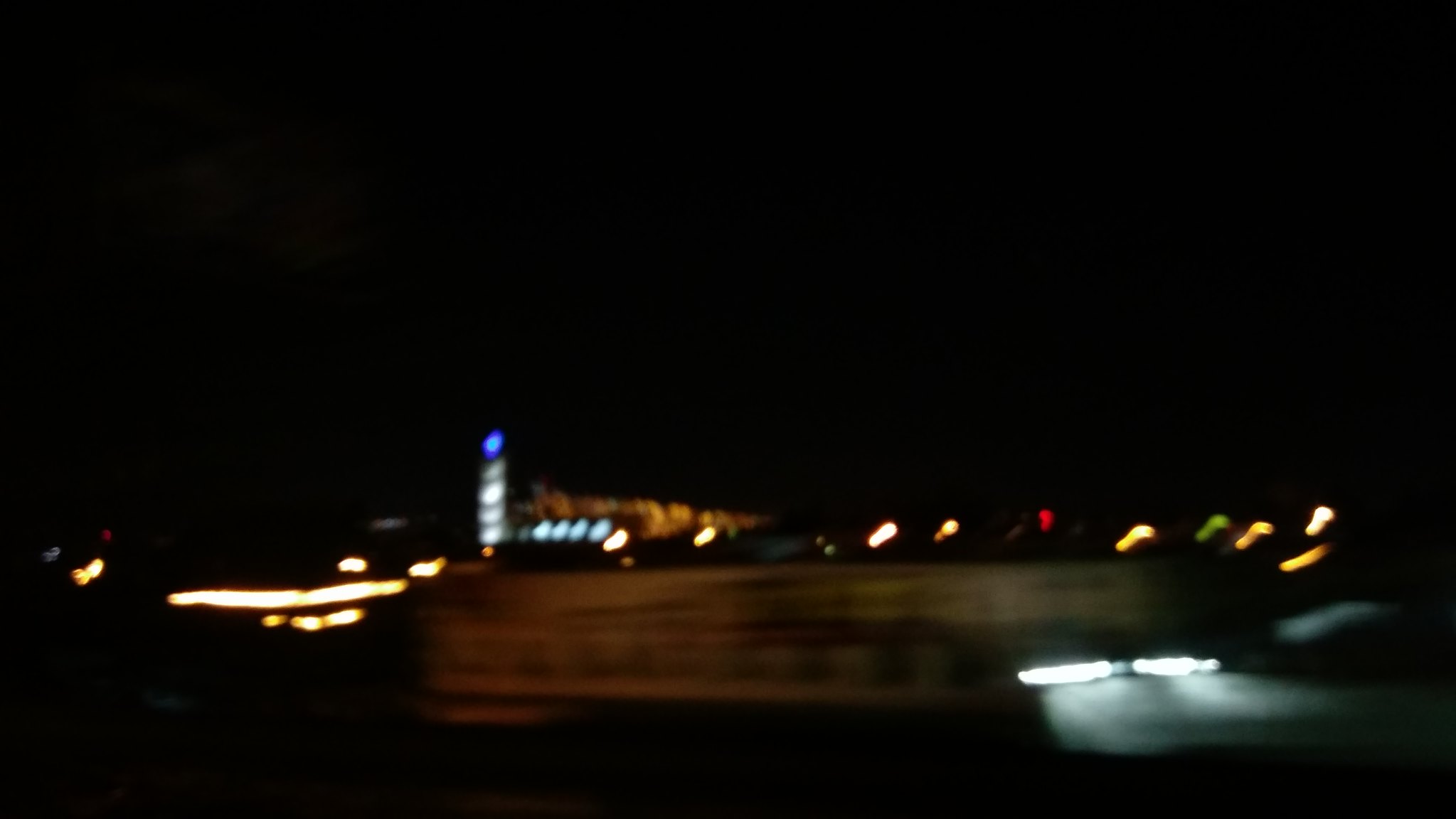A blurry, nighttime photograph taken from a distance, potentially depicting a boat. The image features two bright white horizontal lights in the lower-right corner. Above these lights, several small dots of varying colors are visible, forming a scattered pattern. The lights include, from right to left, yellow, white, yellow, green, yellow, and red. Additionally, a solitary blue light is positioned just left of the center of the image.